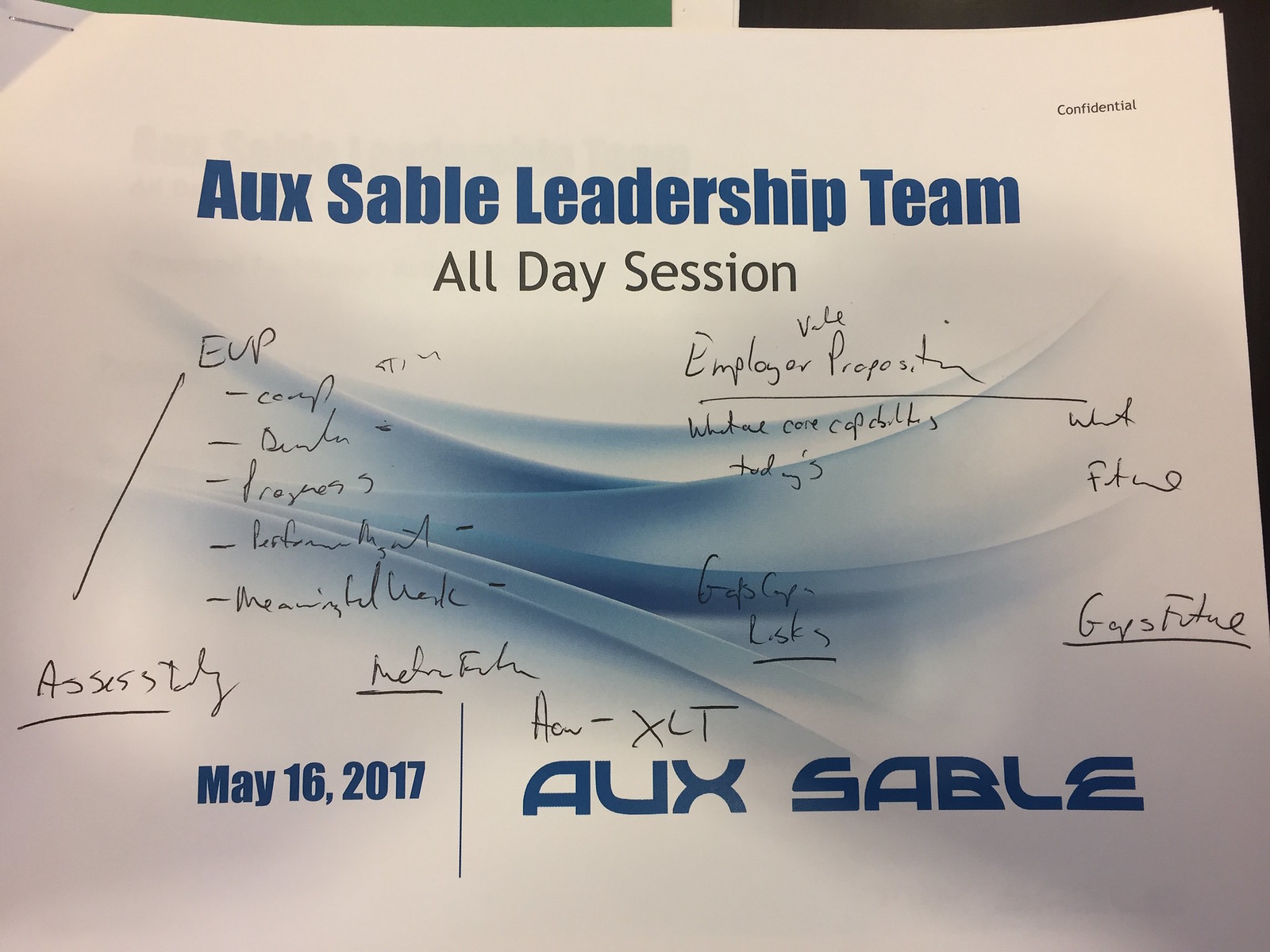This image depicts a detailed and filled-out notepad from the Aux Sable Leadership Team's all-day session held on May 16th, 2017. At the top, centered in blue letters, the heading reads "Aux Sable Leadership Team," with "All Day Session" written in smaller black letters below it. The white sheet features a decorative background with blue swirly and curved designs. To the top right corner, the word "Confidential" is printed in small letters.

In the middle portion of the page, handwritten notes are organized into two columns. The handwriting is somewhat difficult to read but includes terms such as "Employer," "Proposition," "Capabilities," "Meaningful," "Assembly," "Gaps," and "Future" along with "UEP" and "Employee Position," suggesting a brainstorming or discussion session. Towards the bottom, a thin blue vertical line divides the date "May 16, 2017" on the left from "Aux Sable" to the right.